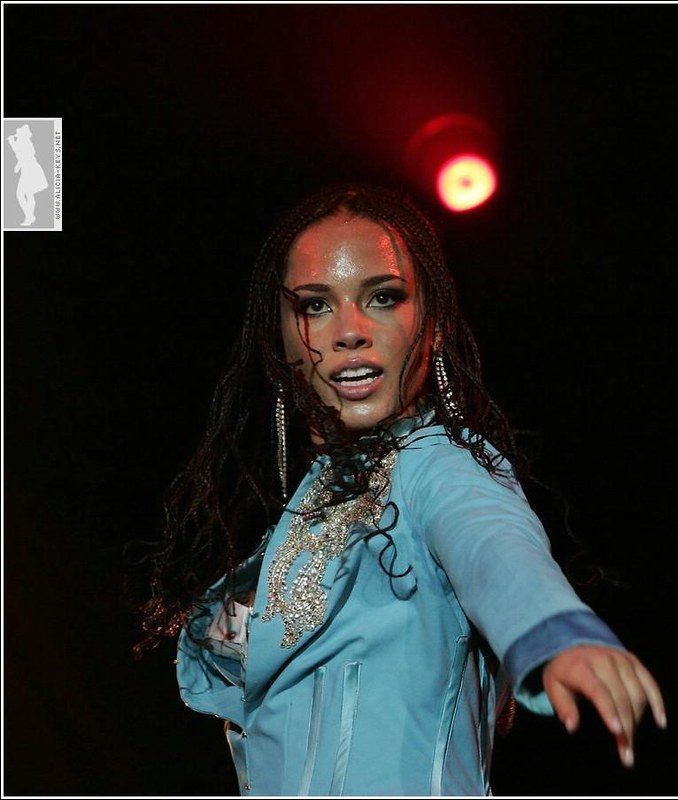In the photograph, an African-American woman is captured mid-performance, either singing or gesturing towards an unseen audience. She wears a striking light blue jacket adorned with an ornate silver bespeckled lapel that elegantly extends towards her neck. Her long braided hair or weave is intricately styled with decorative beads, adding to her vibrant presence.

A spotlight beams down on her, accentuating her expressive features and the dynamic posture of her left arm, which is extended towards the camera, suggesting a powerful connection with her audience. Her facial expression is intensely focused, indicative of her deep engagement in the performance.

In the upper left corner, a white silhouette of a woman singing into a microphone adds a thematic element to the image, reinforcing the context of a musical performance. The woman’s outfit further consists of dark blue sleeves that complement her light blue jacket, creating a visually cohesive appearance. Every detail, from her meticulous hairstyle to her expressive hand, contributes to the arresting energy and vivacity captured in this moment.